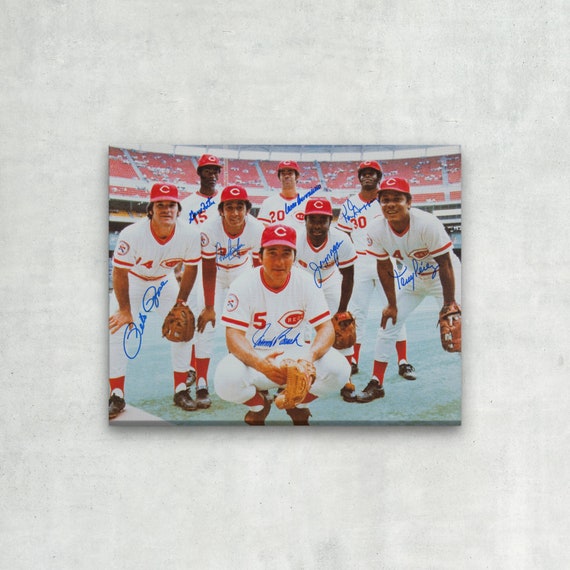The image shows a small keepsake photo, approximately 4x6, lying on a plain white surface. The photograph features a baseball team, possibly the Chicago Reds, composed of eight players wearing white uniforms with red lettering. Each player dons a red baseball cap with a white 'C' on the front. The lineup has one player squatting in the front, four players stooping behind him, and three standing at the back. The uniforms have red numbers on the right chest, red stripes on the sleeves, and are completed with red socks and brown shoes. Each player holds a baseball glove in their left hand. Notably, each player has signed their name above their image in blue pen. The photo is taken in a stadium, evident from the stadium-style seats and some visible fans in the background.